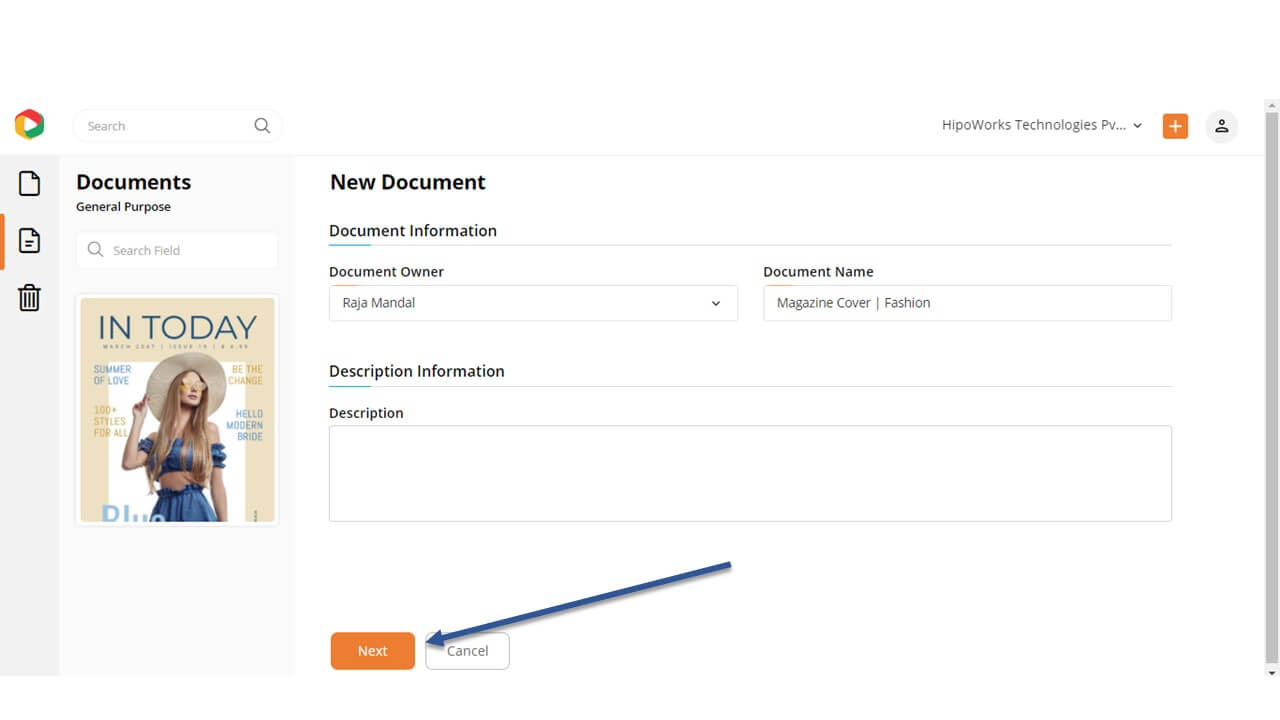This is a detailed screenshot of an app interface with a clean, white background. At the top, the Google Drive icon is prominently displayed next to a small search bar. Below this, three distinct icons are listed: a highlighted Documents icon labeled "General Purpose," followed by a paper icon, and a trash can icon.

Under the "General Purpose" section, another search field is visible, accompanied by a detailed image resembling a magazine cover. The magazine cover features a thick, cream-colored border and, in blue letters at the top, the text "In Today." The cover prominently displays a blonde woman with long hair, wearing a blue crop top and skirt, accessorized with a large summer hat and sunglasses.

Various text elements are scattered around the woman: on the left, "Summer of Love" in blue and "100+ Styles for All" in yellow; on the right, "Be the Change" in yellow and "Hello Modern Bride" in blue. Centrally located in dark letters are the words "New Document."

Below the image, the document information is detailed, listing the document owner as Raja Mondale. The document, aptly named "Magazine Cover Fashion," has further description details available under "Description Information."